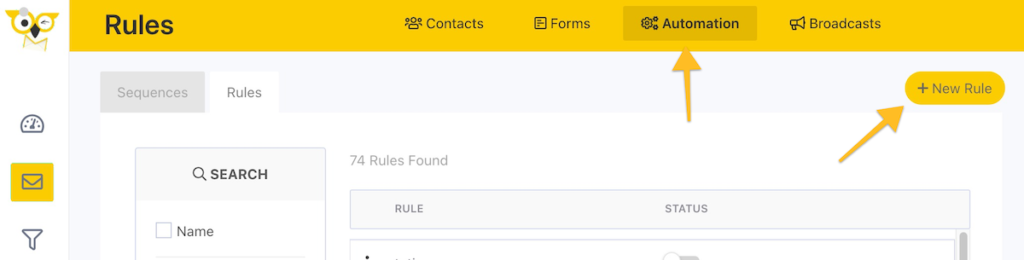Screenshot of a company website highlighting the rules section. The header features a golden-yellow menu bar with options such as "Rules" (displayed prominently in bold black text), "Contacts," "Forms," "Automation," and "Broadcasts." To the left, there's a quirky owl icon wearing glasses and winking, nestling near what looks like a Google-themed 'M' logo, suggesting some affiliation with Google. Directly below the header, a navigation button labeled "New Rule" is adorned with a plus sign. Additionally, menu items like "Sequences" and "Rules" are visible. The side menu includes various icons such as a barometer, mail icon, and funnel, likely representing different functionalities. On the right, the main content area has a white background interrupted only by golden-yellow bars. It showcases a search bar with text indicating "74 rules found," and visual arrows point to areas labeled "Automation" and "New Rule," demonstrating the user interface elements related to rule creation and management.